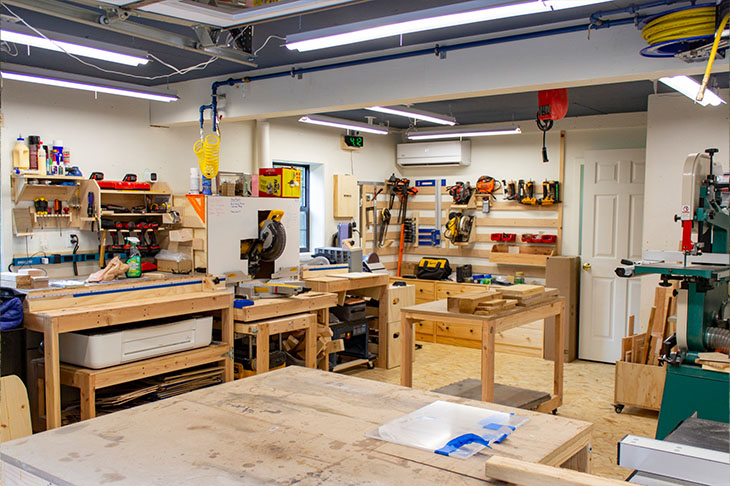This photograph showcases an exceptionally well-organized workshop, likely located in a garage. Wooden tables and workbenches are scattered throughout the space, each holding a variety of tools. The tools are meticulously stored on the walls and under tables, including saws, drills, screwdrivers, and other power tools. There are multiple sets of tools, reminiscent of a well-equipped high school woodshop. The floor is also wooden, adding to the extensive use of wood in the space. Fluorescent light bulbs provide bright overhead lighting, illuminating the entire area. Additional details include scrap pieces of wood, cleaning materials, a prominent green cleaner, a wall-mounted clock, an air conditioning unit, and a ventilation vent. The meticulous organization and the sheer number of tools indicate that the owner has invested significant time and care into maintaining this busy and well-stocked workshop.